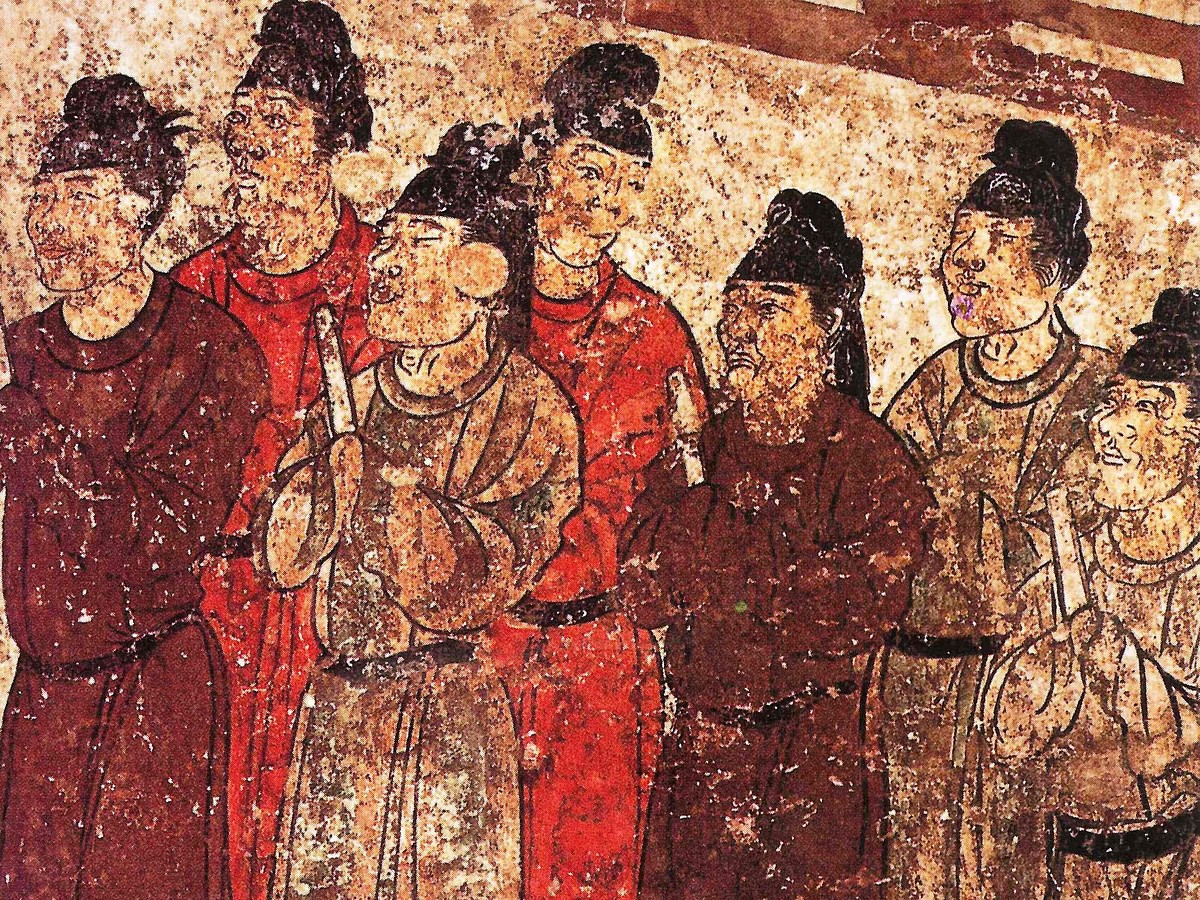The image depicts an ancient, degraded painting on a beige, textured wall, likely made of stone or cement. The overall scene features seven Asian men standing in a row, traditionally dressed in long robes that vary in color from dark brown to maroon, red, and striped patterns. Their hair is styled in buns while some strands cascade down their backs. Four men in the front appear to be holding long, rectangular white objects. The figures are interacting with one another, some wearing smiles and others with closed eyes, exuding a sense of camaraderie. The background is a distressed light tan with specks of dark brown and black, accompanied by brown accent lines in the top right corner resembling a laddering effect. This painting reflects an authentic piece of Asian traditional art, now heavily worn and chipped over time.